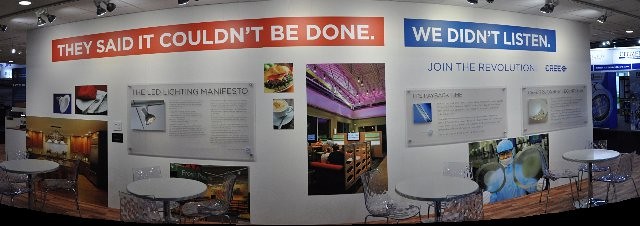The image depicts the interior of a modern cafe, characterized by four circular tables, each surrounded by three to four clear, translucent chairs. The cafe appears well-lit, with a white ceiling equipped with lights that illuminate the space. Dominating the scene is a large, wide white divider wall adorned with various images, photographs, and texts. On the top left of the wall, a red rectangular banner with white capital letters reads, "THEY SAID IT COULDN'T BE DONE", while on the top right, a blue rectangular banner with white capital letters states, "WE DIDN'T LISTEN". Beneath these banners are several boxes containing text and images, including an individual in medical scrubs. Also visible are pictures of a burger and a restaurant. The wall appears to detail accomplishments or milestones, with the overall design contributing to a theme of innovation and success. The space extends further into the background, adding depth to the room.